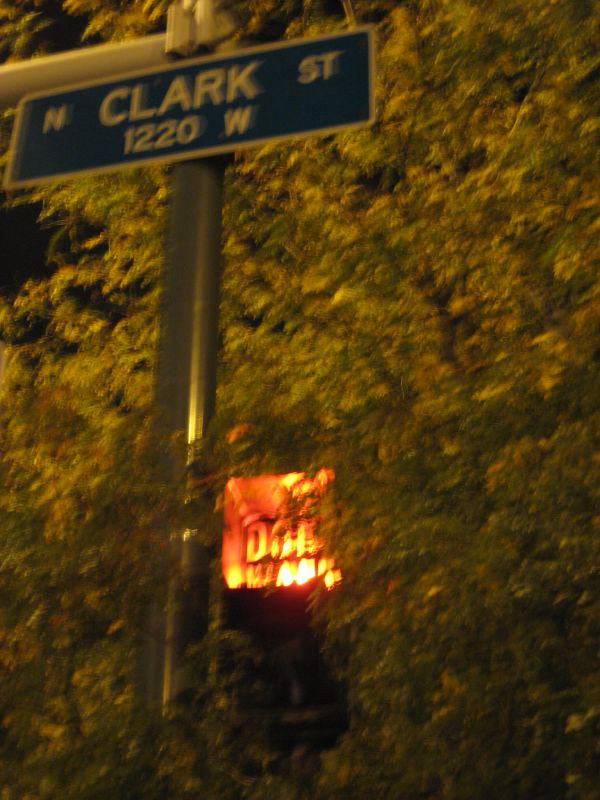This photograph captures an outdoor scene centered around a street sign. The sign itself is mounted on a dark-colored pole. To the right of the image, there is a square-shaped "Walk/Don't Walk" signal. The signal is illuminated in red, clearly displaying "Don't Walk." Higher up on the pole, there is a green street sign with white outlines and text that reads "N. Clark Street, 1220 W," indicating the location as North Clark Street at the 1220th West Block.

Extending from the pole towards the left and near the top of the image, a silver bar pole is visible. The background is filled with trees, their leaves lush and abundant, partially obscuring the "Don't Walk" sign and a branch crossing in front of the pole. The scene is dimly lit from above, suggesting that the photo was taken at night. The dark background further complements this nighttime setting, contrasting with the vivid green foliage.